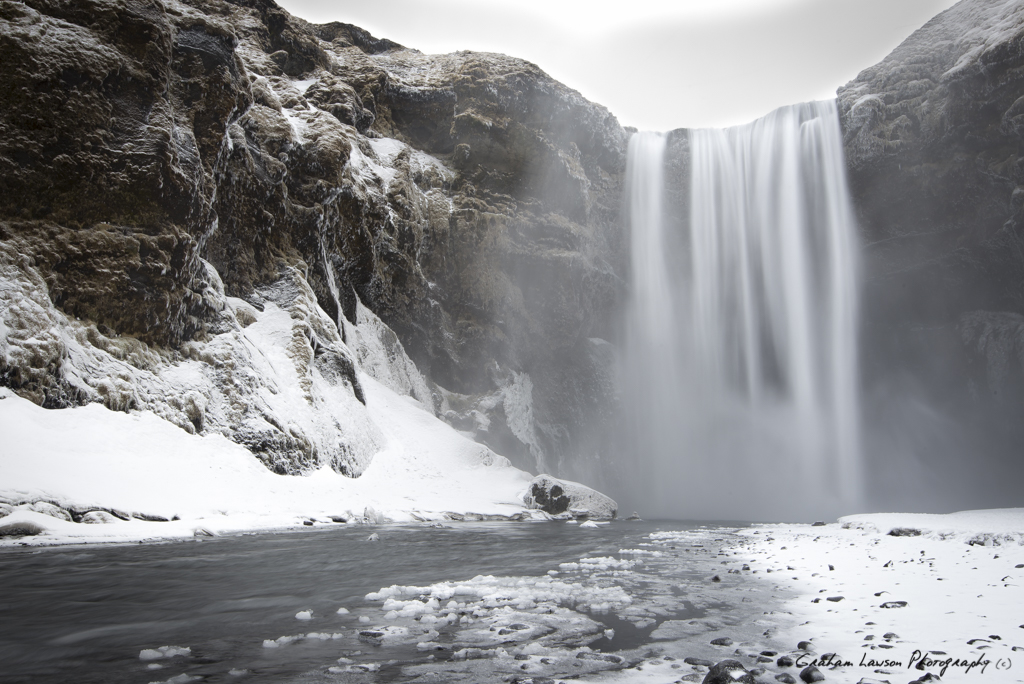In this captivating black-and-white photograph by Graham Lawson, a majestic waterfall cascades over a rugged, snow-covered cliff into an icy stream below. The landscape is predominantly wintery, with snow blanketing the ground and bits of brown and gray rock peeking through. Smaller rocks are scattered in the foreground, partially submerged in the frigid water. As the powerful water hits the stream, a visible mist rises, adding an ethereal quality to the scene. The sky above is heavily overcast, creating a moody backdrop. The right side of the image features more of the cliffs and snow-covered areas, contrasting with the left side's rocky terrain. In the bottom left corner, the fine print reads "Graham Lawson Photography (C)," indicating the photographer's copyright. This image beautifully captures the serene yet powerful essence of a winter waterfall, making it a perfect piece for wall decor.